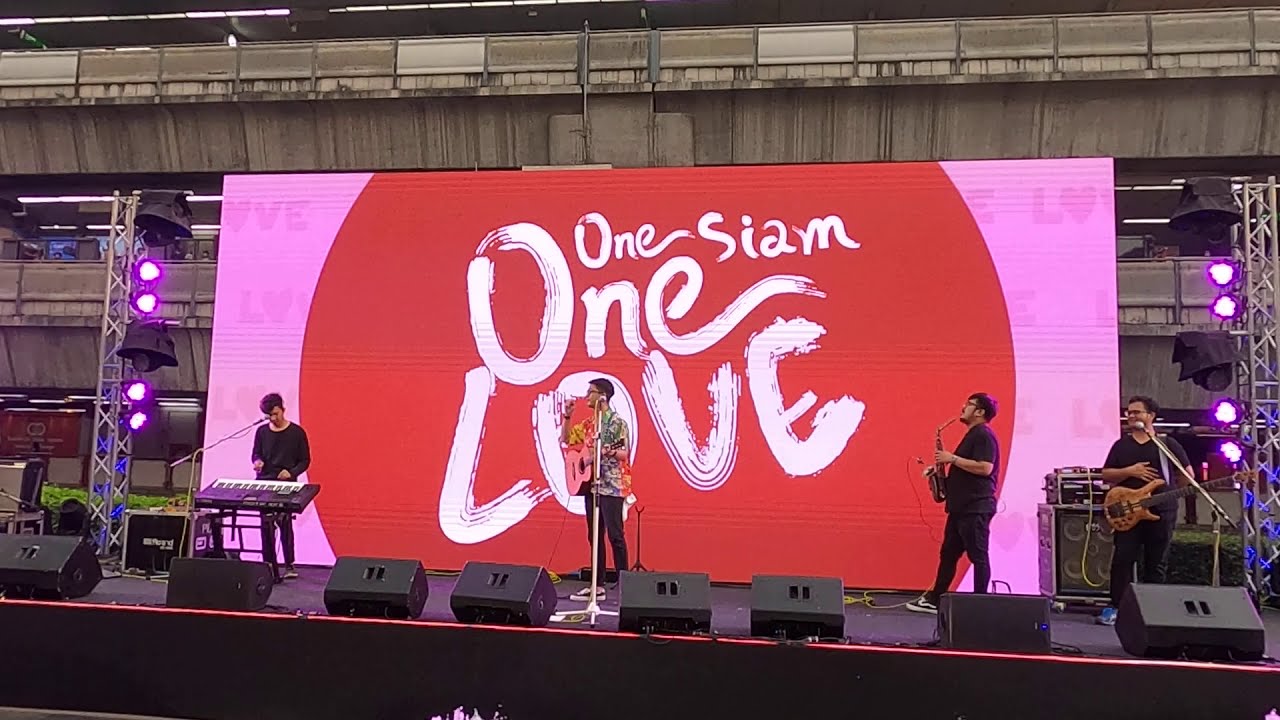The image captures a band performing on a stage set against a backdrop featuring a large red circle with the white text "One Siam One Love" on a pink background. The stage, viewed at a slight angle, has a dark black floor with edges highlighted by thin red lines. Along the front of the stage are multiple black speaker boxes, and the structure behind the stage includes brownish-tan walls with open viewing areas on two floors. Vertical metal beams on either side of the stage have pairs of purple lights shining from them.

On stage, four band members are performing. From left to right: the first musician, dressed entirely in black, is playing the keyboard with a microphone stand in front of him. Next, the guitarist, wearing a brightly colored Hawaiian shirt, stands at the center, looking towards the keyboardist and equipped with a white mic stand. To his right, a saxophonist, also dressed in black, is positioned, looking left. On the far right is the bass player, adorned in black like the others, with a microphone in front of him and what appears to be an amplifier behind him. The scene captures the lively ambiance and setup of the band's performance.